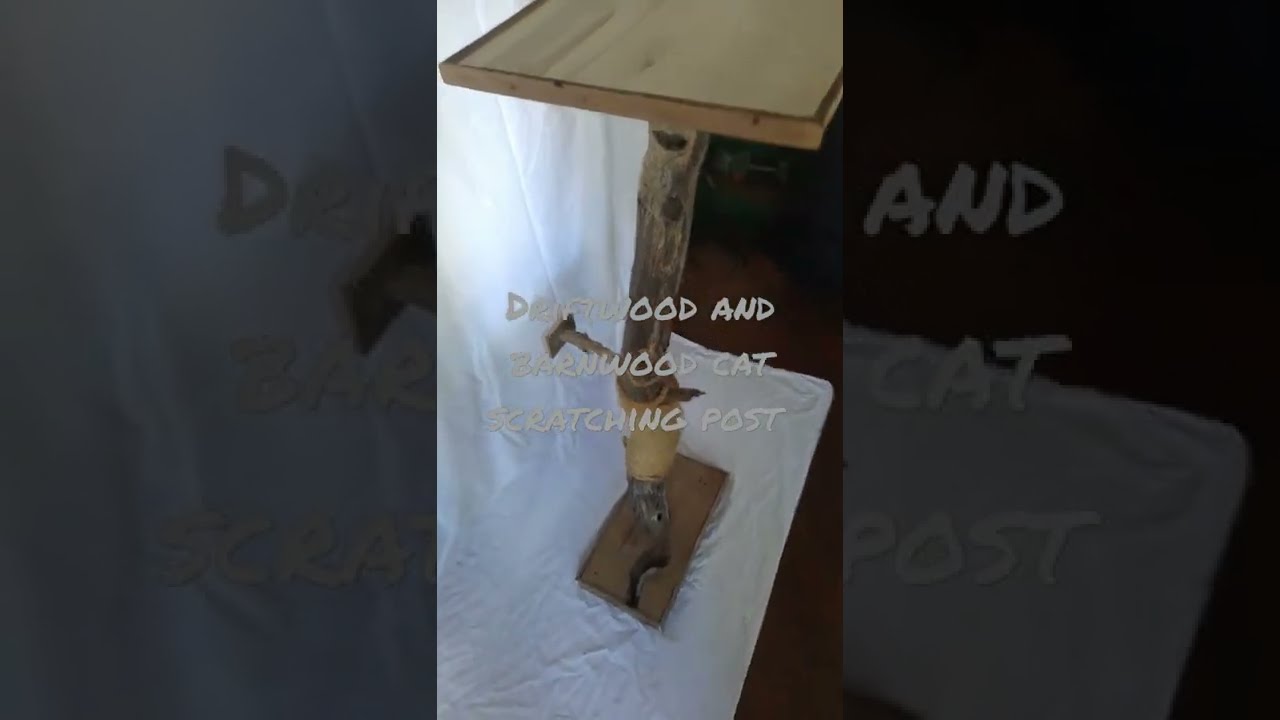The image is divided into three vertical sections, with the outer sections featuring a darkened close-up of the middle section. The central portion showcases a wooden cat scratching post placed on a white cloth that extends across the floor. The post consists of a light beige driftwood upper section and a darker barnwood lower section, connected by a wooden log. The setting appears to be indoors, with the post prominently positioned in the center of the image, partially cut off at the top. Additional elements include wood flooring and a curtain draped over the floor to the left. The text, in a cream handwritten font, reads “Driftwood and Barnwood Cat Scratching Post,” positioned centrally over the image. The style resembles a screenshot from a mobile app like TikTok or Instagram, featuring a mix of white, off-white, brown, black, and gray colors.